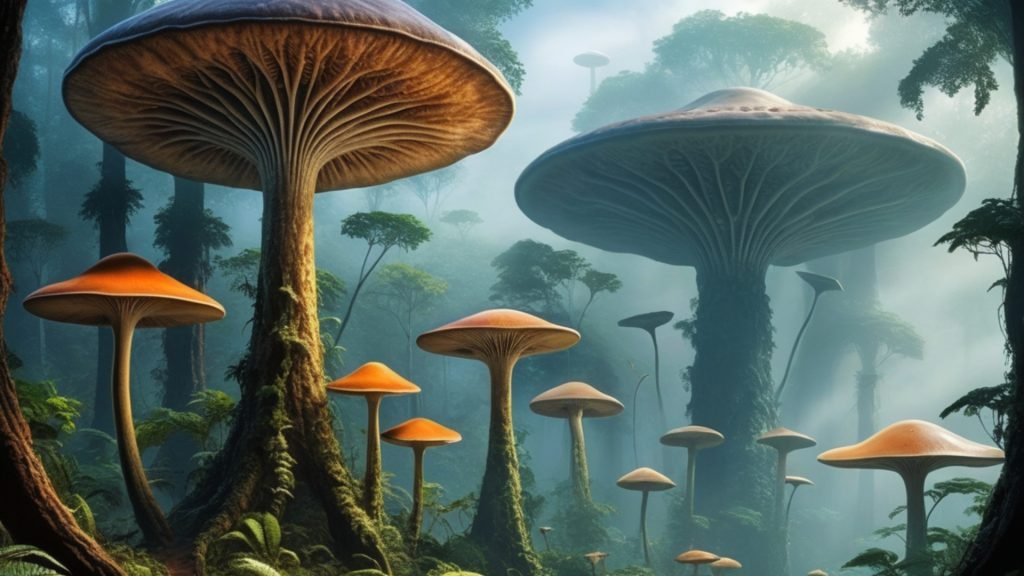The image is a captivating, computer-generated painting of a surreal landscape, likely an alien planet, featuring an otherworldly forest composed of giant mushrooms rather than traditional trees. The scene is enveloped in a dense, cool fog, lending a mystical and somewhat eerie atmosphere. Dominating the composition are two colossal mushrooms taking up each half of the image. These mushrooms, with their thick, branch-like bases resembling tree trunks, are covered in lush moss and ferns. Their caps are intricately veined and detailed, with striking orange and white hues. Surrounding these towering fungi are clusters of smaller mushrooms and an array of exotic greenery, which include rainforest-like trees that add to the forest's richness. The foreground presents a sharp focus on the detailed textures and vibrant colors of the mushrooms and accompanying plants, while the background fades away into a mist, creating an enchanting, dreamlike quality.